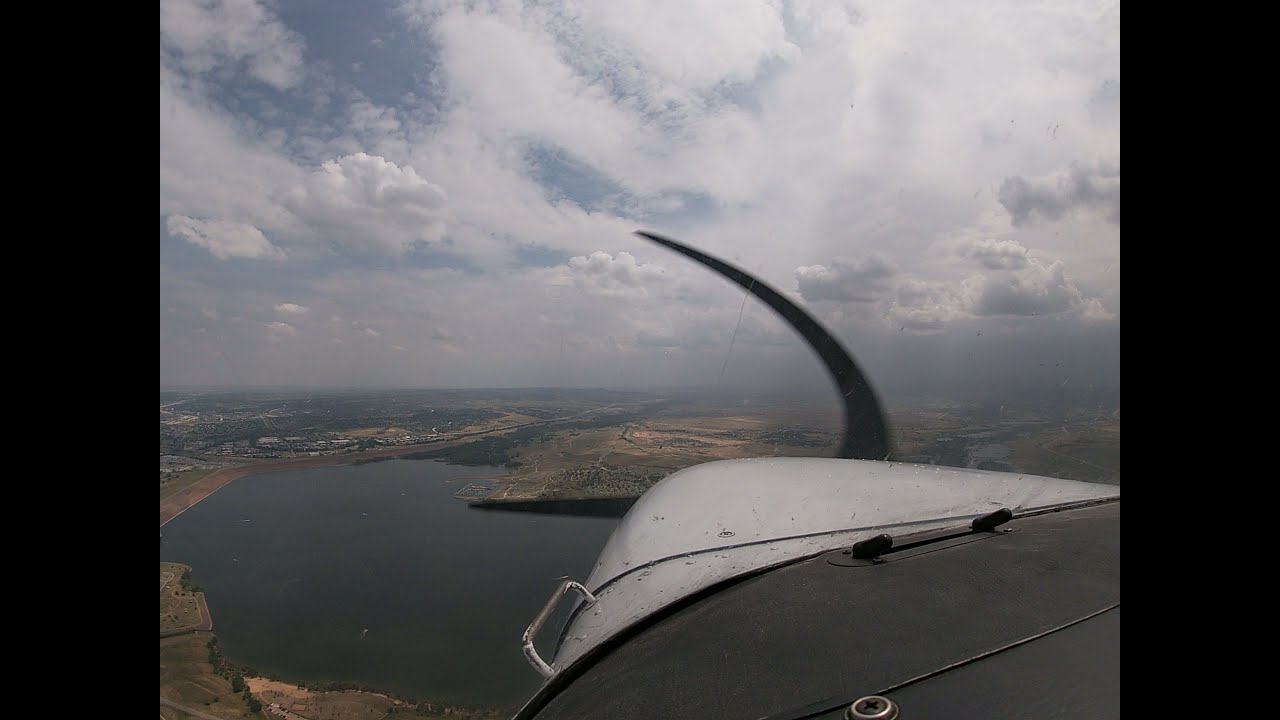This image is taken from the window of a small dual-engine propeller plane, revealing a detailed aerial view below. The foreground prominently features the white metal wing, which transitions to black near the tip adorned with a large crescent-shaped, black fin wrapping around it. There's also a metallic golden circular object and a handle attached to the black section of the wing. The wing and the spinning propeller, blurred by motion, subtly frame the landscape below.

The scenery beneath includes a round-shaped lake resembling a race track, indicating its unique curvature. Surrounding the lake, a small town is noticeable with distinct houses and a few office-like buildings scattered along the shoreline. The lake's water appears dark green, dotted with small boats. The land stretches into rural expanses covered in green trees that look almost black from this high vantage point.

The sky above is dramatic; the horizon transitions from dark, rain-laden clouds on the right to partially cloudy areas on the left where patches of blue peek through. The scene suggests that the plane is flying below the dense cloud cover, possibly preparing for landing, given the detailed ground visibility and the proximity to the lake and town below.